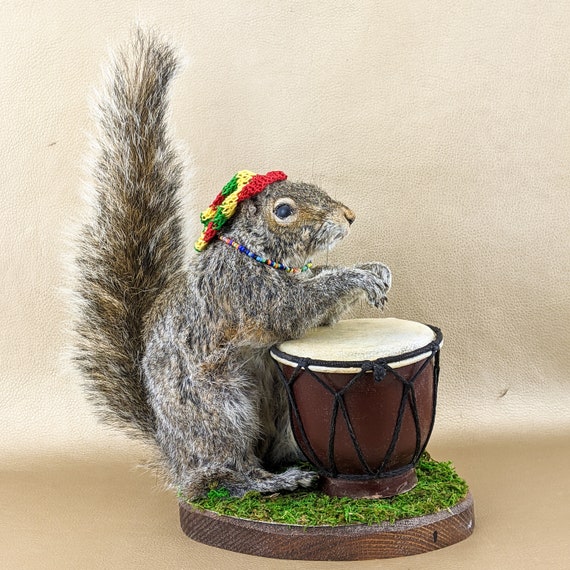The image showcases a detailed and lifelike representation of a squirrel, possibly taxidermied or expertly crafted to appear realistic. The squirrel is standing on its hind legs on a wooden pedestal covered with fake green grass, situated against a white background. It faces the left side of the photograph, with its fluffy tail sticking straight up into the air. The squirrel's arms are raised, with its front paws resting on a bongo drum that features a white top, brown sides, and is decorated with black rope. Notably adorned, the squirrel wears a multicolored Rastafarian hat—composed of red, yellow, and green patches—and a beaded necklace with an array of different colors. This image captures a whimsical diorama of a squirrel seemingly engrossed in playing the bongo drum.